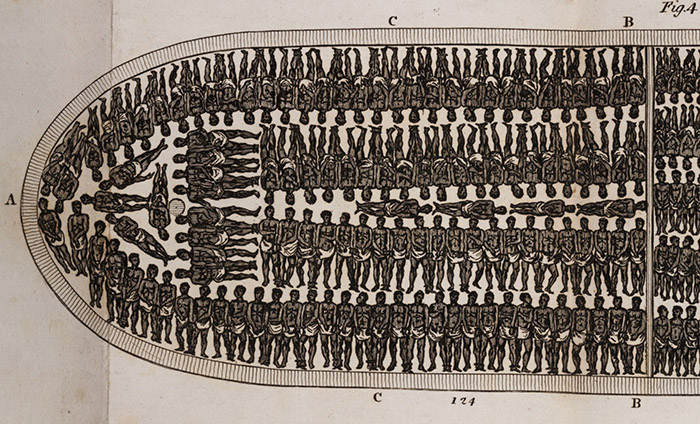This black-and-white line drawing illustrates the harrowing conditions aboard a slave ship. The ship's hold is densely packed with male slaves, lying shoulder to shoulder, with their arms crossed and bodies compressed in such a way that they have no room for movement. The drawing shows detailed organization: slaves are arranged end-to-end and head-to-toe, occupying every inch of space. Along the outer edges of the image, various letters and numbers are marked, including 'A,' 'B,' 'C,' and the sequence '1, 2, 4,' as well as 'figure 4' in black text at the top right. The vessel's interior is depicted as a rounded structure with a straight middle section, suggesting confined, claustrophobic quarters. Some slaves appear to be outfitted with simple white loin cloths. The layout showcases slaves in multiple orientations: some standing along the edges and many more lying down in tight sequences throughout the middle. The rear of the ship is also shown to be heavily crowded, illustrating the inhumane conditions endured during the Middle Passage.